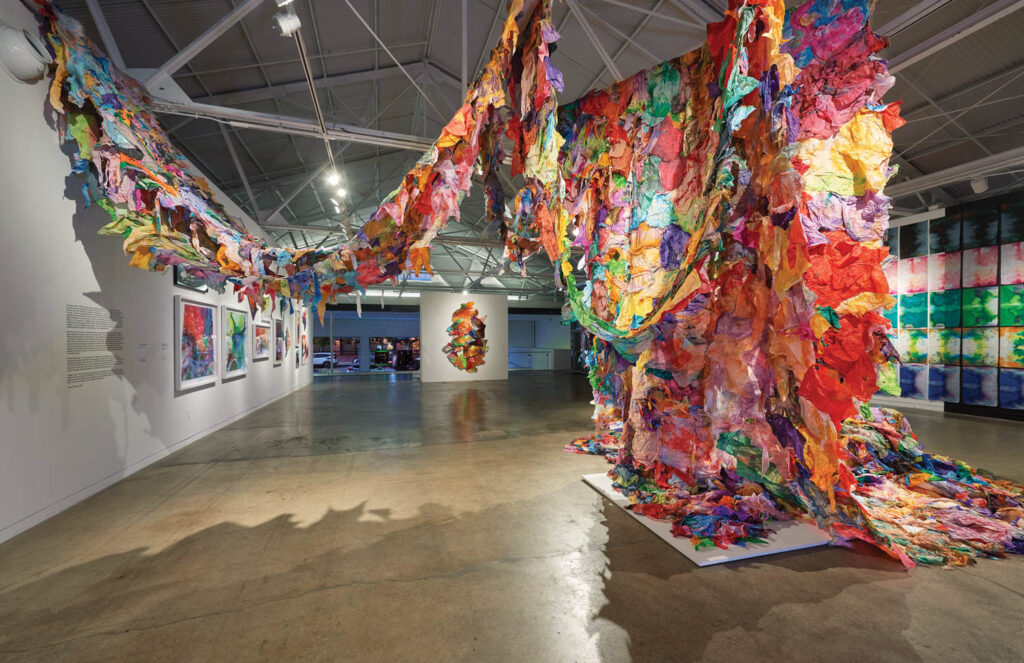The photograph captures an art gallery featuring a striking installation as its focal point. This central piece is an elaborate fabric sculpture, composed of assorted colorful fabrics—green, orange, yellow, red, blue, and purple—that cascade from the ceiling, drape along one gallery wall, and pool dramatically on the floor. The gallery itself is spacious with concrete floors and white walls adorned with various brightly colored, framed watercolor artworks. In the background, the area opens up to other sections of the gallery, revealing additional vibrant pieces. The ceiling installation's dynamic arrangement and vivid hues stand out against the gallery's minimalist setting, offering a rich texture that contrasts with the surrounding artworks and polished brown floor. Nearest to the camera, there is a set of descriptive text on the wall, presumably providing context to the exhibit, enhancing the viewer's experience of this immersive and vibrant display.